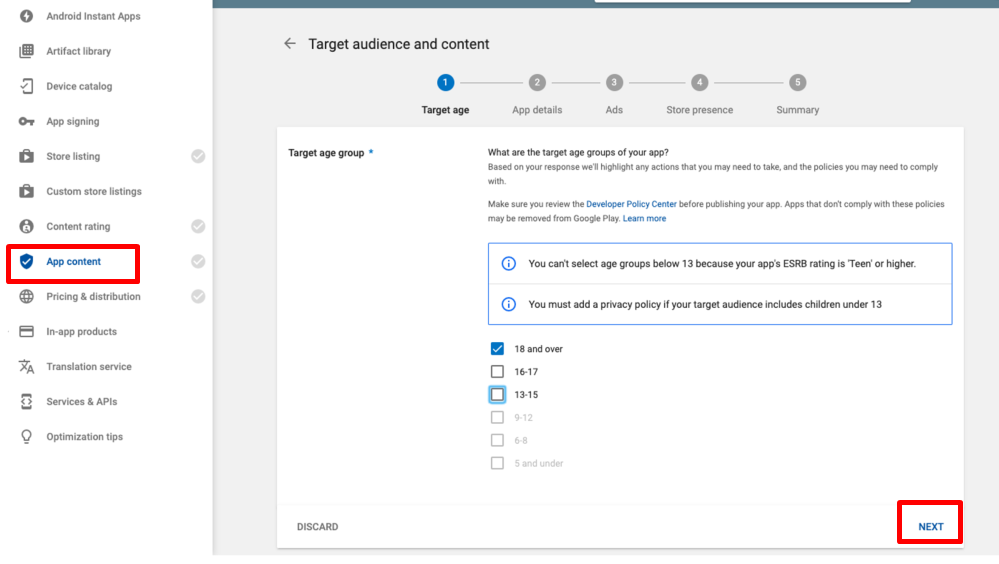The image depicts a detailed page from a digital platform, likely a developer console for an app store, dealing with the setup of an app’s target audience and content classification.

On the left side of the page, there is a vertical menu with a white background and clickable list items in gray. The menu items from top to bottom include:
1. Android Instant Apps
2. Artifact Library
3. Device Catalog
4. App Signing
5. Store Listing
6. Custom Store Listing
7. Content Rating
8. App Rating (highlighted in blue with a red outlined box)
9. Pricing
10. Distribution
11. In-App Products
12. Translation Service
13. Services & APIs
14. Optimization Tips

On the right side of the page, in the bottom right corner, there is another red outlined box with the word “Next” in blue, serving as a navigation button.

The main content area at the top of the page is titled "Target Audience and Content" and features graphical elements, including several connected circles representing different sections:
1. Target Age (colored blue)
2. App Details
3. Ads
4. Store Presence
5. Summary

Below this header, there is a section explaining the "Target Age Group," outlined within a white box. The section describes the process of selecting the appropriate age groups for the app.

Further down, within a blue box, there are details about the ESRB rating and checkable options for different age groups. These options include:
- 18 and over (highlighted in blue)
- 17 to 16
- 13 to 15
- Additional lower age groups.

This comprehensive layout provides developers with the necessary tools and guidance to categorize their app correctly based on the target audience and content ratings.